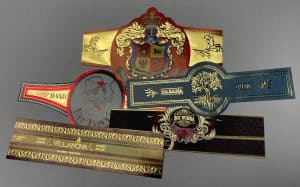The image depicts an array of five ornate, decorative objects, each suggesting a semblance to championship belts often associated with boxing or wrestling. On the bottom left lies a gold ruler, while beside it to the right is a mainly black, wide belt adorned with golden inlay. Moving upwards, the second item is a black velvet rectangular band featuring a distinct badge in its center. Further up, there is a blue belt accentuated by a golden tree emblem at its heart. The fourth object is notable for its prominent coat of arms, flanked by two gold lions with additional gold eagles on either side. The topmost belt is particularly elaborate, showcasing a grand coat of arms and intricate golden and red designs. Collectively, these items exhibit an assortment of colors and intricate patterns on a grayish backdrop, each piece varying in detail and embellishment.